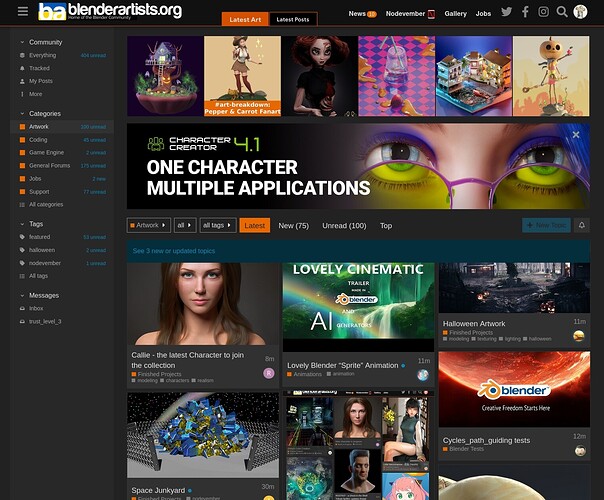This is a detailed description of the character-building page for Blender Artists at blenderartists.org. The page appears to be designed for gamers and character creators, prominently advertising "Character Creator 4.1" with the tagline "One Character, Multiple Applications." 

At the top of the page, there is a stock image of a woman with deep-set eyes accentuated by purple eye shadow. She is wearing yellow, round-rimmed glasses, which lend her a distinct look. Above her image, there are several character images presumably created by users. On the far right, there is a character resembling a jack-o'-lantern, possibly inspired by Tim Burton, holding either a guitar or a weapon. Next to it is an image capturing three adjacent hotel or condo buildings.

Another character showcased is a knight with a seemingly squiggly lance, creating an optical illusion that makes it ambiguous whether he is stepping on a lake or involved with spilling liquids resembling blue and gold substances. Additionally, there's an image of a 16th-century explorer or conquistador, hinting at character avatars that can be crafted with historical backgrounds.

Towards the bottom of the page, users are presented with more options, including an image of a woman named Callie, the latest character in the collection. She has long brown hair and deep-set eyes, gazing intently at the viewer. Her image is cropped just below the neck, making it difficult to discern her attire.

In the middle section, a green box featuring Earth emitting rainbow light in space is present, resembling imagery from Star Wars. It is labeled "Lovely Cinematic Trailer - AI Generated," suggesting a deeper creative avenue for character development. Adjacent to it is a section labeled "Halloween Artwork," likely another resource for character images.

The second row continues the theme with a "Space Junkyard" image designed for character utilization and a "Lovely Blender Sprite Animation" box for creating animated cartoons. The row ends with an outer space scene labeled "Cycles Path Guiding Tests," another creative tool for enhancing or adding to user-created characters or storylines, reinforcing the site’s affinity for sci-fi imagery.